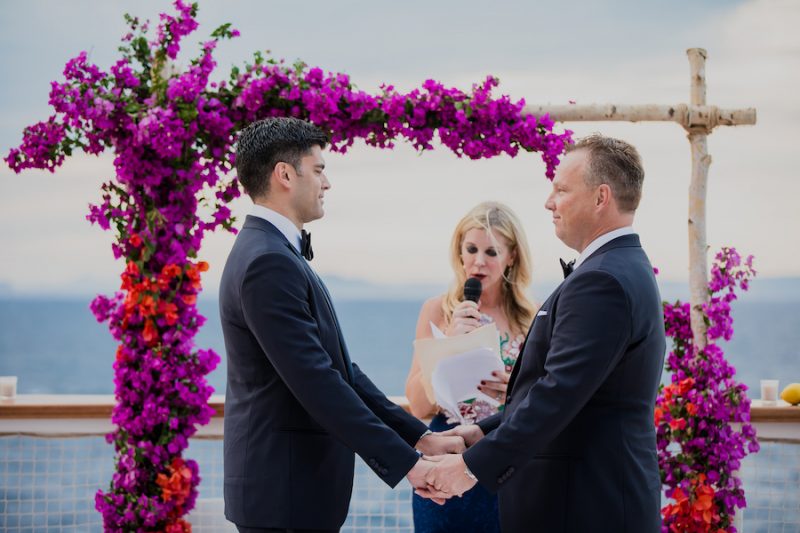This photograph captures a touching wedding ceremony between two men, set against a stunning backdrop by the ocean. Both grooms are wearing dark suits—one described as navy blue and the other black—with white shirts and bow ties. They are standing on a platform with a railing and wire fencing, holding hands and gazing lovingly at each other. The groom on the left, who is taller with a chiseled and rugged look and darker hair, stands opposite the shorter groom on the right, who has lighter, thinning hair and a slightly fuller figure. They are deeply in love, as evident from their tender expressions.

The officiant, a blonde woman, stands before them with a microphone and stack of papers, speaking to a larger crowd. Behind her is an exquisite floral arch described as made from birch wood poles arranged in a square shape. The arch is adorned with a cascade of vibrant purple and red flowers, especially dense at the top left corner, gradually thinning out to reveal the wooden structure on the right. Additional details include a fence and a lemon with a glass of something resting on the beam of the fence in the background. The serene water behind them adds further to the enchantment of the scene.